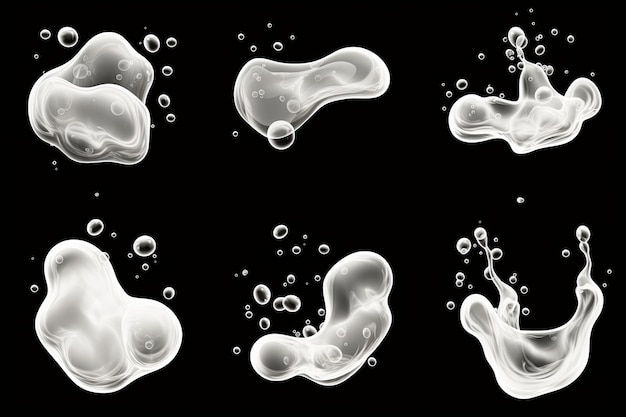The image showcases a detailed graphic illustration of six large, white water blobs set against a stark black background. These blobs exude a sense of fluidity, as if they are suspended in water or captured in zero gravity, exhibiting an ethereal, floating quality. Each blob, surrounded by smaller bubbling droplets, differs in shape and form, adding to the dynamic nature of the scene. Arranged in two rows of three, the top left blob resembles a hat or a triangular shape dotted with tiny bubbles. To its right, a bubble elongated to mimic a video game controller or a dog bone, and the final one in the top row appears splashed, with a triangular center and knob-like ends. In the bottom row, the left blob exhibits a V shape, likened to the palm of a hand, while the central one is curved and oblong, reminiscent of a couch. Lastly, the bottom right blob is U-shaped, highlighting the splashing effect of water, with numerous smaller bubbles around it. The overall composition is devoid of any text, focusing entirely on the intricate and captivating details of the water blobs against the plain background.